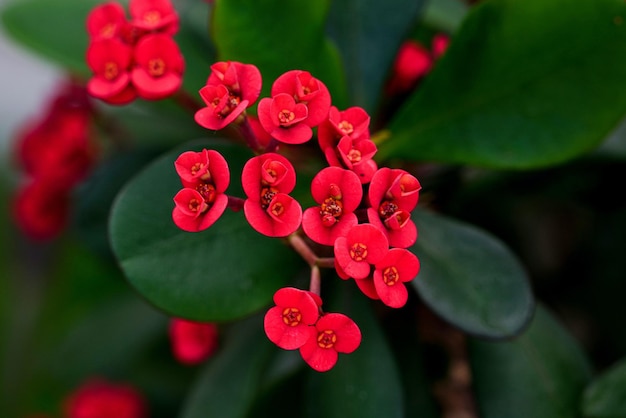This is a close-up photograph showcasing a fascinating red flower with a unique structure. The central flower splits into two smaller flowers within the same base, creating a repetitive spiral pattern of cylindrical forms. Surrounding the vibrant red blooms, which have hints of fuchsia and lighter red star patterns, are dark green, oval-shaped leaves that might remind one of rubber plant foliage. These leaves contrast beautifully with the cluster of flowers and are interspersed with lighter green shades in the blurred background. The reddish-orange stems with splotches of green add to the medley of colors. Beneath the central cluster of red flowers are two prominent dark green leaves, while more leaves can be seen scattered throughout the front and blurred sides of the image, suggesting an abundant, thriving plant. The photograph, taken in bright midday light, captures multiple clusters of these striking flowers, focusing primarily on the central group while hinting at more in the background.